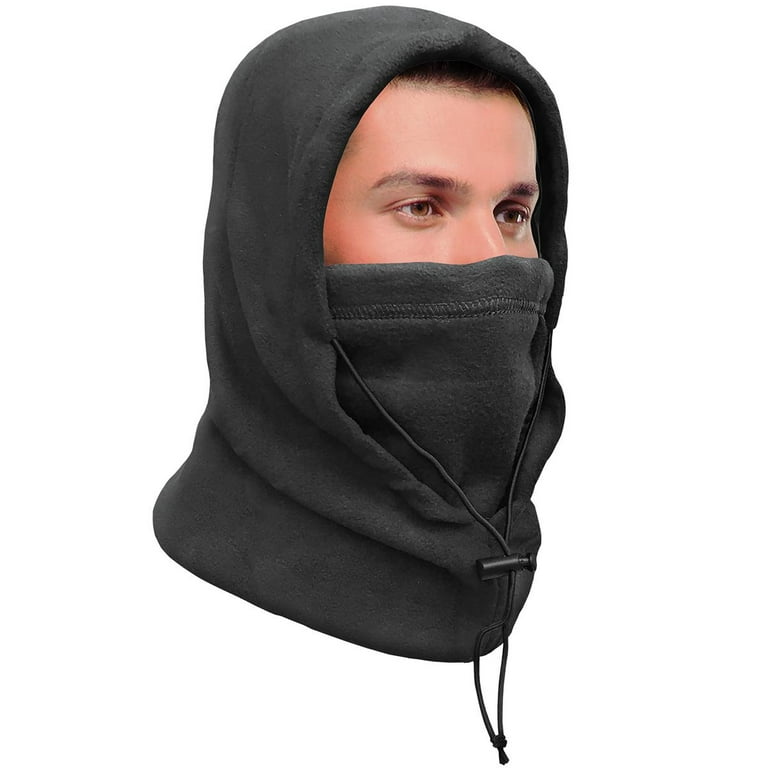This image features a young Caucasian man with short dark hair and dark eyebrows, partially obscured by a dark gray hoodie and mask combination. The top part of his face, from his forehead to the bridge of his nose, is visible, while the hood and attached mask cover the rest. The mask, which appears hemmed about an inch from the end, is integrated into the hood but its attachment method is not clear. The hood, which is dark gray like the mask, includes black drawstrings with a small plastic piece that can be adjusted to tighten or loosen the fit. The young man is facing three-quarters to his left, making his right side more visible to the viewer. The entire scene is set against a pure white background, emphasizing the dark hues of the hood and mask.